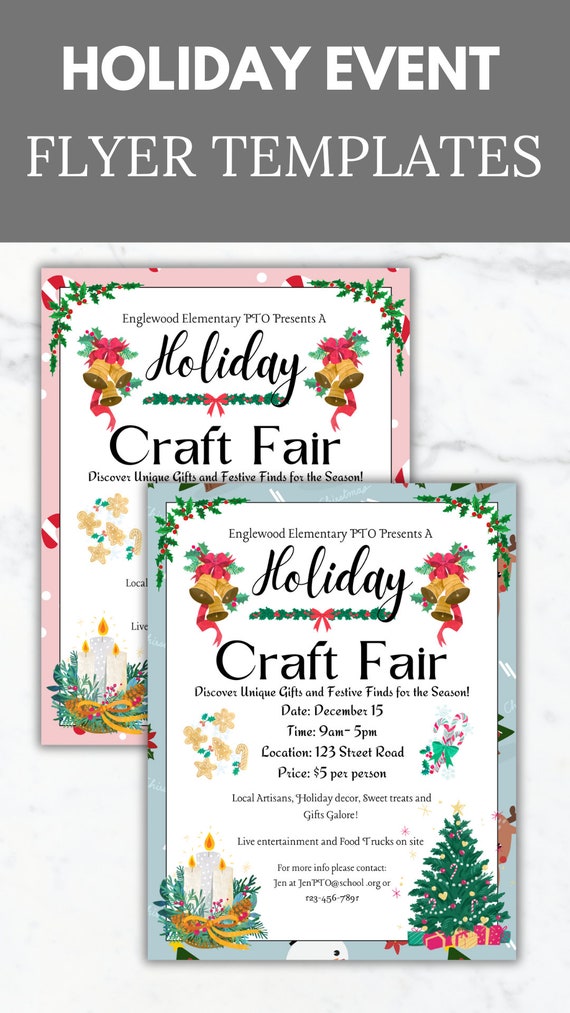This portrait-mode promotional ad for holiday event flyer templates features a gray banner with white lettering at the top, stating "Holiday Event Flyer Templates." Below the banner, two overlapping example templates are displayed against a white marble background. The top template, clearly visible, is gray and reads: "Englewood Elementary PTO presents a Holiday Craft Fair. Discover unique gifts and festive finds for the season!" Key details include:

- **Date:** December 15th
- **Time:** 9 a.m. to 5 p.m.
- **Location:** 123 Street Road
- **Price:** $5 per person

The flyer promotes offerings from local artisans, holiday decor, sweet treats, and abundant gift options. It also highlights live entertainment and food trucks on site. Further information can be obtained by contacting Gen at genpto.school.org or a placeholder phone number 1-2-3-4-5-6-7-8-9-0.

Decorative elements include cartoon images of a Christmas tree, a group of lit candles, bells with red ribbons, and candy canes. The bottom left-hand corner of the templates features candles, while the bottom right-hand corner displays a Christmas tree. Additionally, holly wreaths with red bows adorn the section just beneath the main announcement. The templates are available in pink and light blue variations.